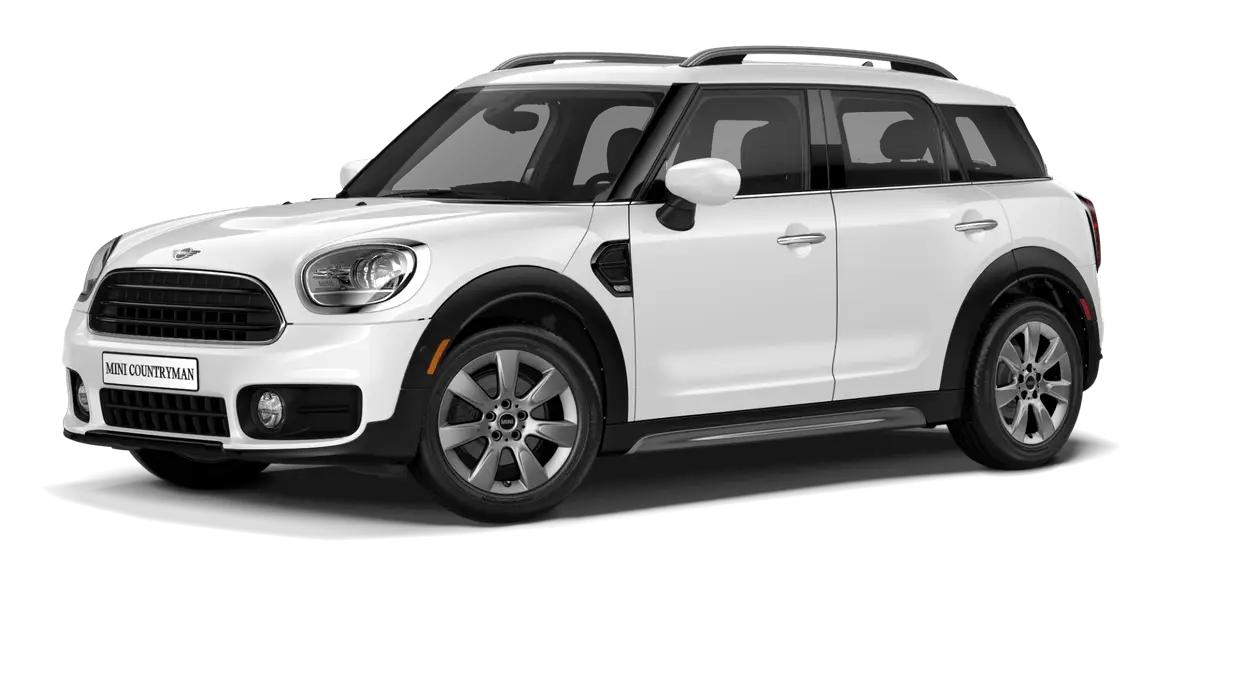The image features a pristine white Mini Countryman set against a solid white background, likely used as a stock photo for marketing purposes. The car is positioned with its front pointing to the left. Prominently displayed on the front license plate is the name "Mini Countryman," alongside the hood ornament logo. The vehicle includes notable details like two headlights and additional spotlights at the lower front. Black trim accentuates the car's design, while the windows are slightly tinted black. The car has four doors, with two visible silver door handles on the side shown. The white body sports silver wheel coverings and an overall sleek, new appearance. Atop the vehicle is a luggage rack, perfect for securing cargo. Shadows beneath the car add depth to the otherwise stark background. Parts of the black-colored interior, including the steering wheel, front and back seats, passenger seat, and rearview mirror, are faintly visible through the windows.